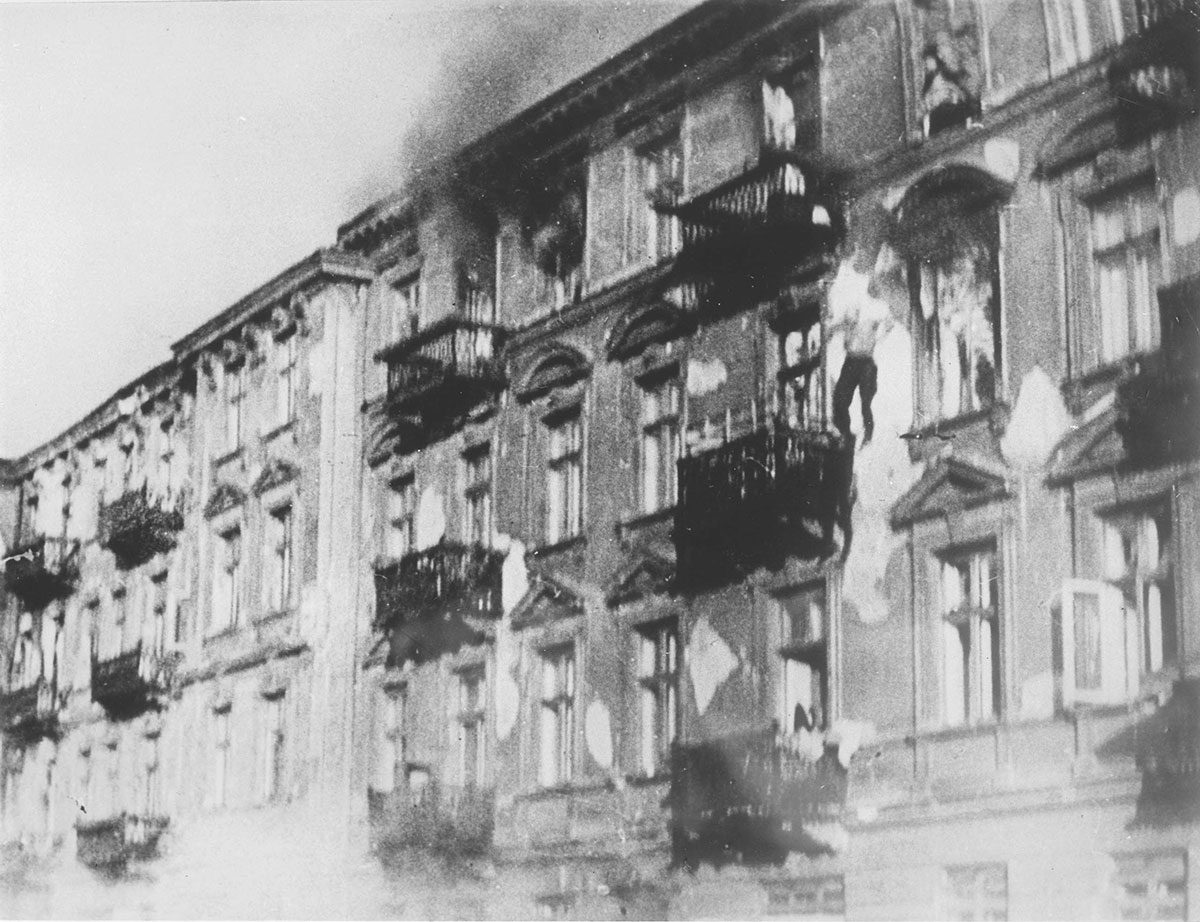In this grainy, black-and-white photograph, a distressing scene unfolds among a row of nearly identical apartment buildings, each featuring rectangular windows and occasional balconies. Heavy, dark smoke billows from the upper floors of the central building, suggesting a severe fire. Amidst this chaos, a man, seemingly shirtless and wearing dark pants, is captured mid-jump from what appears to be the third or fourth floor, likely driven by the fear that the inferno would consume him. His arms are outstretched, and he looks down toward the ground. The exterior of the buildings shows signs of blackening, reinforcing the severity of the fire. The overall composition and elements of the scene evoke a palpable sense of urgency and peril.